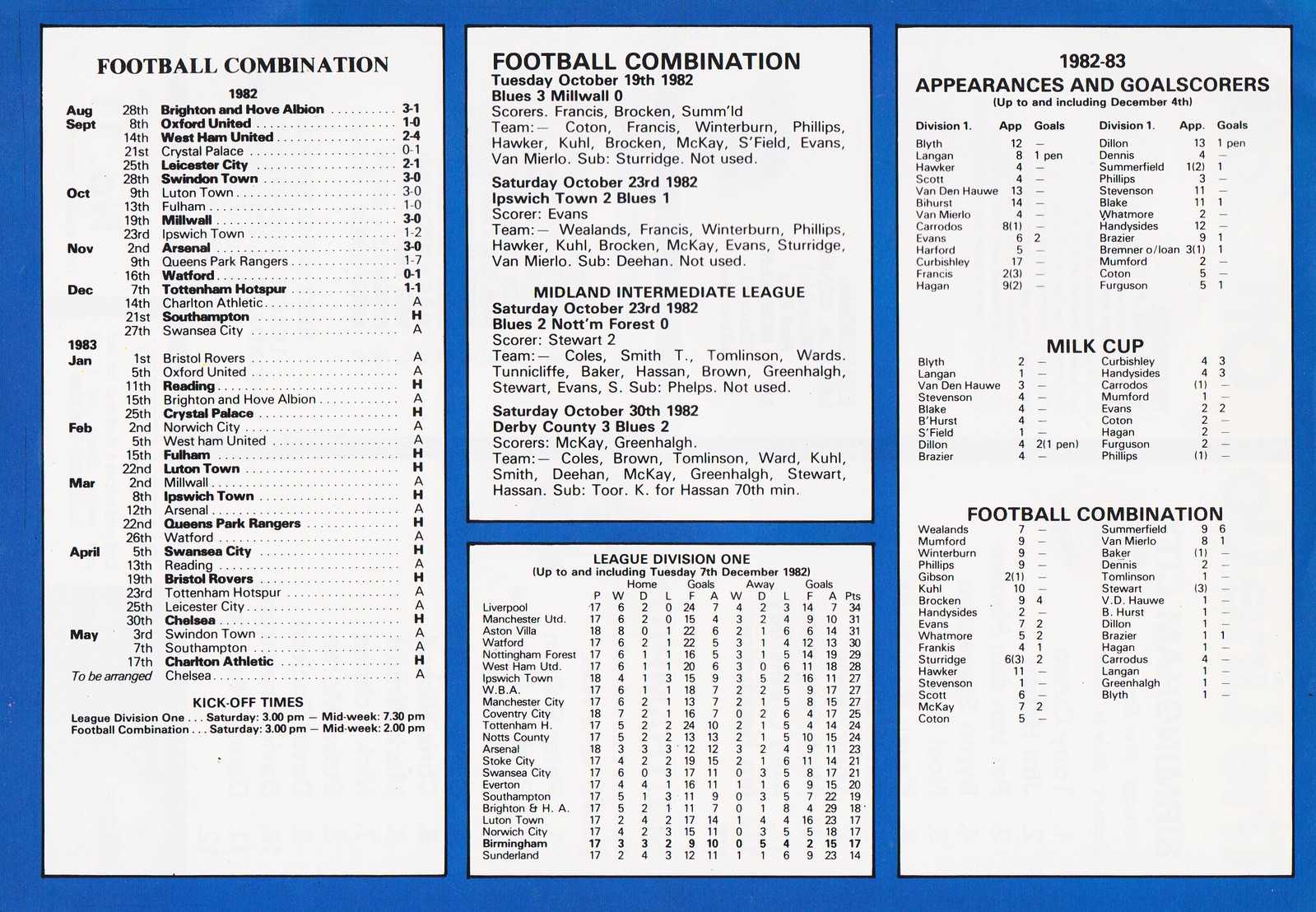The image depicts a detailed sign featuring football statistics and information, likely from England given the mention of teams like Chelsea, Nottingham Forest, Millwall, and others. The sign is divided into four sections, each bordered in blue. The first section prominently displays "Football Combination," repeated in the second section, which is shorter. The third section is labeled "League Division One," listing various players or teams, though the print is small and somewhat difficult to read. The final section heading reads "1982-83 Appearances and Goal Scorers," followed by further details, including "Milk Cup" and "Football Combination."

The information includes dates, scores, and lists of team names and players, providing insights into who favored to win and the specifics of home and away games. The statistics include game dates such as Tuesday, October 19th, 1982, with a match score of Blues 3, Middlewell 6, and another on Saturday, October 23rd, 1982, showing Ipswich down to Blues 1. Player names like Francis, Winterburn, and Phillips are mentioned, alongside detailed game stats and substitutions, offering a comprehensive snapshot of football data from the period.